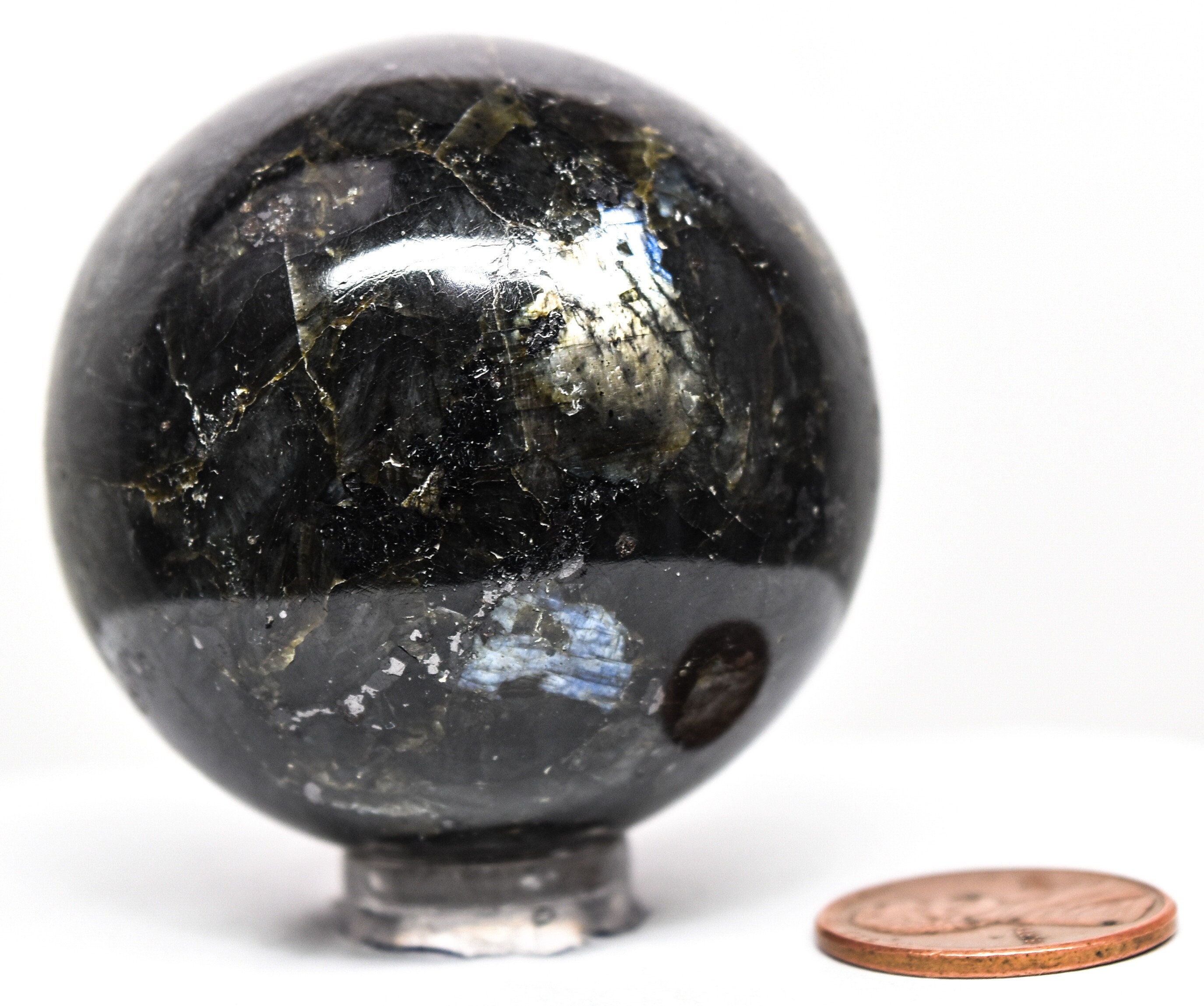The image depicts a close-up of a polished, shiny black sphere, embellished with intricate gold and white streaks, possibly indicating it's a mineral such as onyx or marble. This reflective sphere, roughly the size of a golf ball or perhaps a bit larger, sits securely on a small, finely-cut silver stand, resembling a base or mount. A penny placed to the lower right of the sphere in the photo provides a sense of scale, showing that the sphere is relatively small. The penny, heads up with Abraham Lincoln’s head facing away from the viewer, is shorter than the height of the stand, emphasizing the compact size of the sphere.